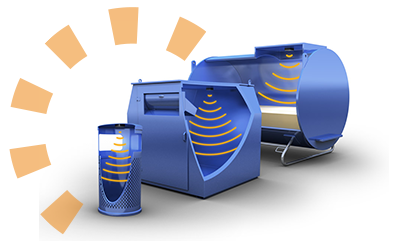The image features a white background and showcases six distinct structures arranged in a circular pattern. On the far right, there is a blue cylindrical object resembling a trash can or dumpster, with yellow lines in the middle that suggest wireless signal waves or radar emissions. Next to it, and more toward the center, there is another similar blue object also emitting radar-like waves. Towards the left, these objects seem to transform into different forms – one resembling a cylindrical tank with an opening and sound waves emanating from the top, while another appears to be a dispenser-like device with a slot for inserting items. In the top right section, there is a tubular structure that resembles a tanning bed, visibly allowing a glimpse inside where the bed is located. Additionally, orange sound waves are illustrated emerging from various points on these objects. Completing the scene, a semicircle on the far left emits orange and yellow beams, reminiscent of sunlight or sound waves, integrating into the overall cohesive theme of emission and reception signals among these diverse and visually descriptive components.